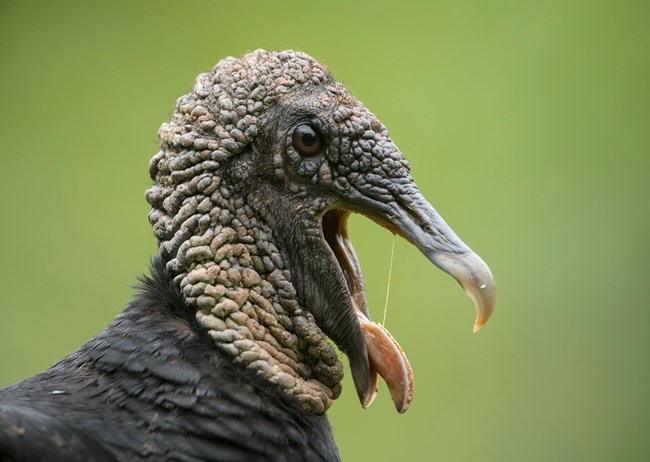This up-close photograph captures a striking image of a bird, likely from the turkey or vulture family, with a partially open beak that reveals a pinkish tongue protruding slightly and glistening with a layer of saliva. The bird, shown in profile, displays a head and neck covered in wrinkled, hard-textured skin of a dark tan or brownish color with a notably curved beak. Its single visible eye is brown, set against a rough, brain-like texture running from its forehead down to its neck. The head and neck transition into short, black feathers visible just below the neck. The background highlights the bird against a pea green color gradient, lighter in the center and darker toward the edges, enhancing the prehistoric appearance of this compelling avian subject.